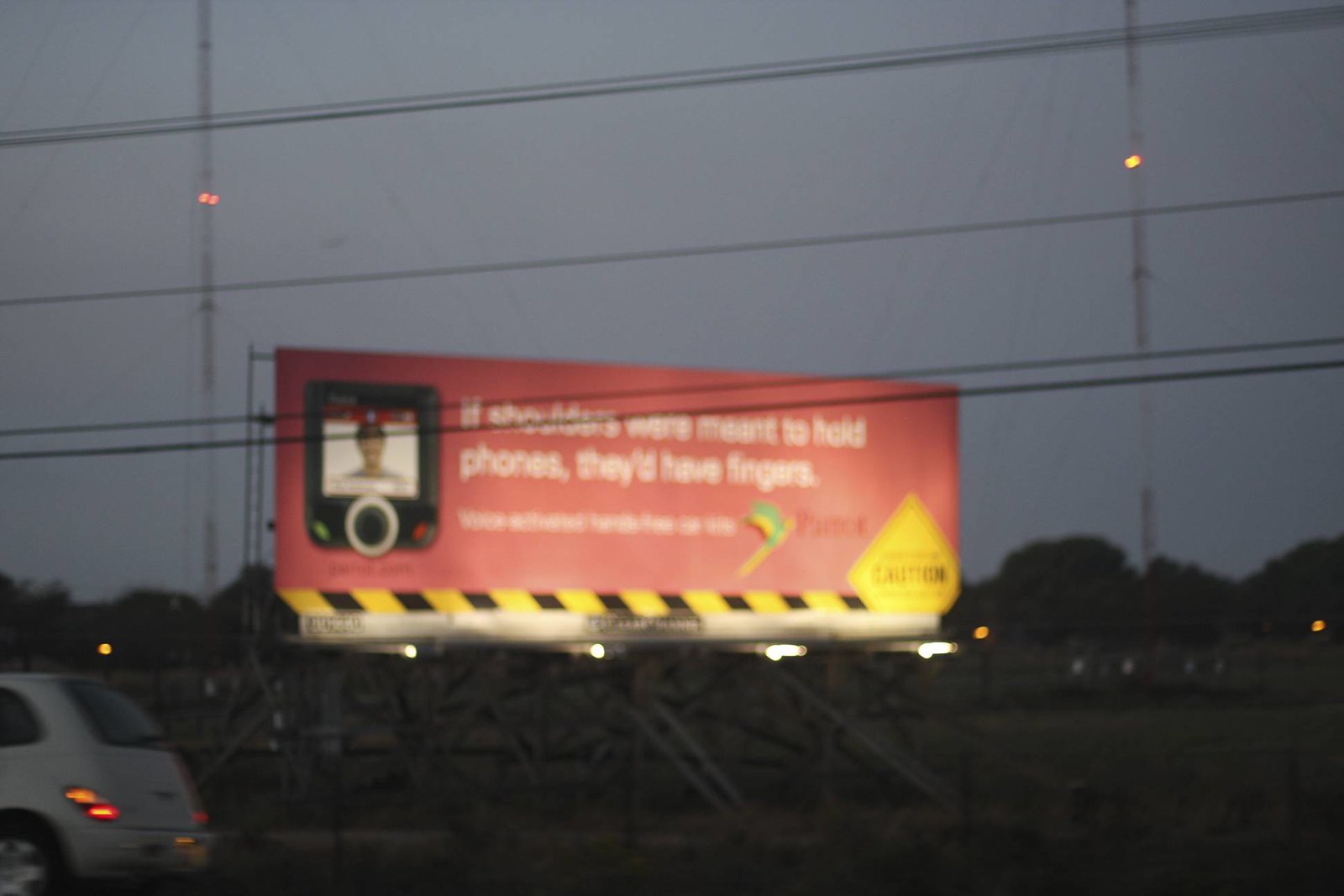This image captures a billboard from the perspective of a car in motion, imparting a sense of active travel. In the background, a PT Cruiser is visible, also driving, adding to the feeling of shared movement. The photo is slightly blurry, enhancing the impression of speed and making some details harder to discern. The billboard features an image of an old, antiquated flip phone, juxtaposing past technological concerns with present-day issues. The text on the billboard humorously suggests that if shoulders were meant to hold phones, they would have fingers, cautioning against the outdated practice of propping phones on shoulders while driving. Below the billboard, a caution sign and caution tape emphasize the safety message. The image evokes nostalgia for a time when distracted driving warnings were simpler, contrasting sharply with today's multifaceted distractions involving social media and smartphone apps.